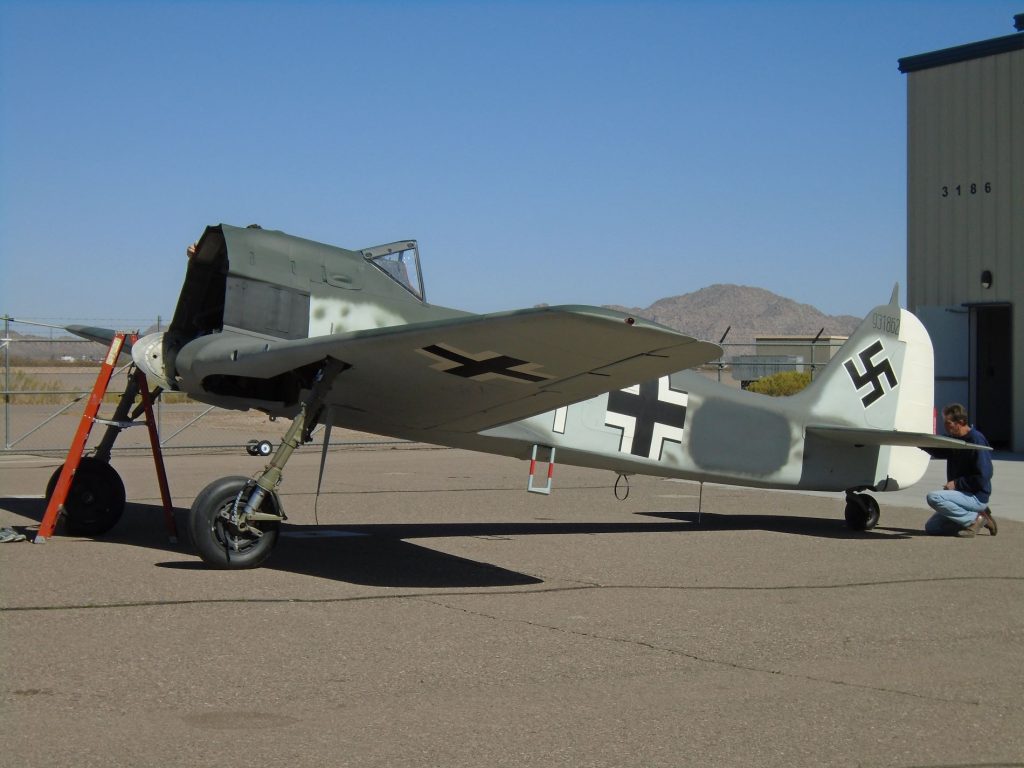The photograph captures a scene featuring a vintage World War II-era German fighter plane, identifiable by its gray fuselage adorned with black-and-white cross symbols on its sides and wings, as well as a black swastika on the tail rudder. The plane, devoid of its engine and cockpit glass, stands on a concrete surface, its right side facing the camera. A lone man, likely in his 50s, donning a blue sweatshirt, faded blue denim Levi's, and brown boots, is kneeling at the tail, apparently working on the rudder area. A ladder is propped next to the left wing, hinting at ongoing maintenance or repair efforts. In the backdrop, a stark blue sky meets a mountainous desert landscape, and a portion of a high industrial building is visible in the upper right corner of the image.